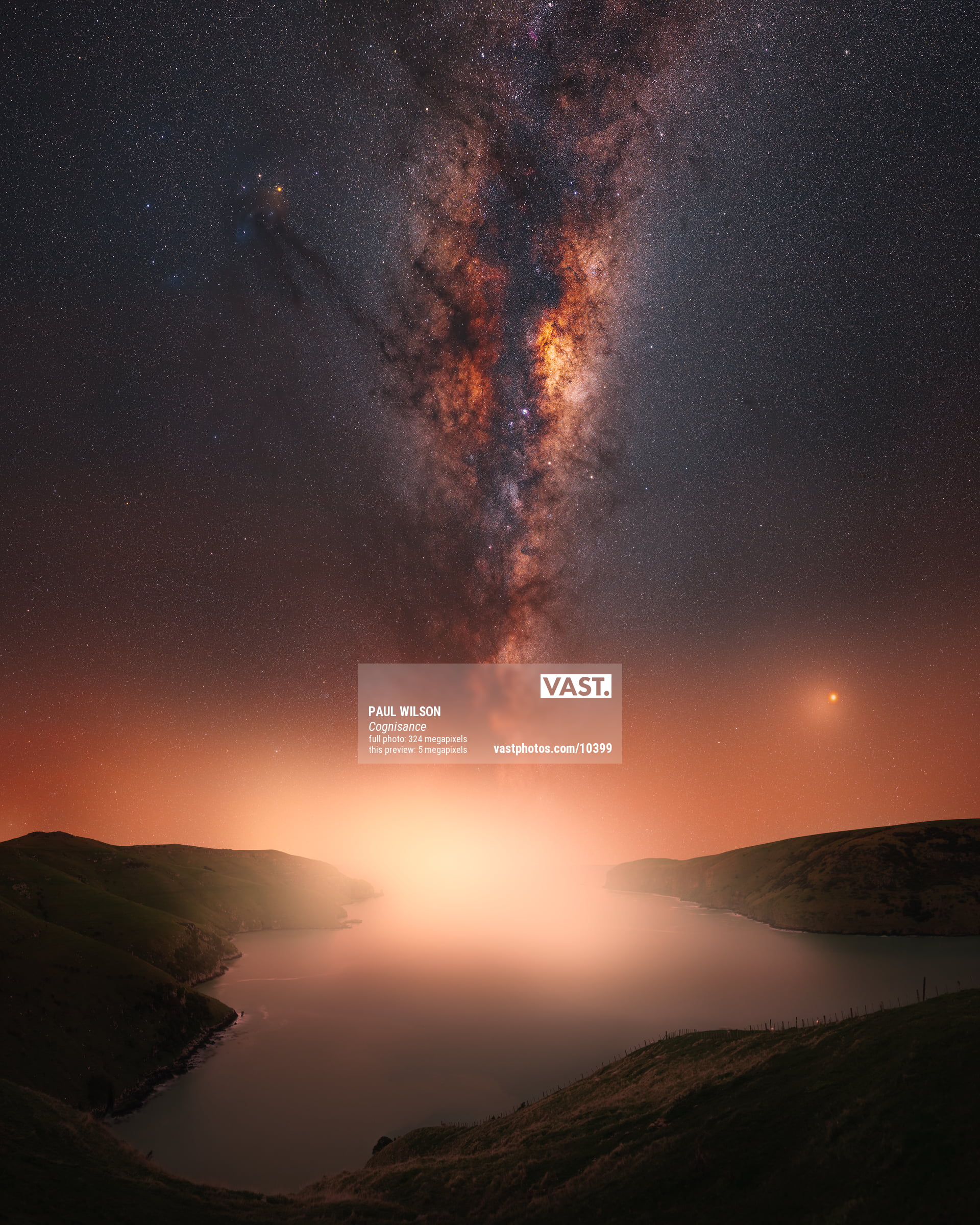This photo captures a breathtaking view of a night sky dominated by the Milky Way galaxy, slicing through the center and displaying millions of stars in various hues of blue, orange, yellow, and purple. The scene overlooks a smooth body of water, likely a lake or bay, flanked by large hillsides on the left and right. The horizon features a bright white light, possibly from a setting or rising sun, which illuminates the water and casts an ethereal glow over the landscape. The sky transitions from an orange hue near the horizon to a darker, star-filled expanse above, with a grayish gaseous column running through the Milky Way.

A semi-transparent rectangle, slightly blurring the background, appears near the center of the image. This rectangle includes solid edges, with "Paul Wilson Cognizance" written inside, and indicates the full photo resolution is 324 megapixels while the preview is 5 megapixels. In the top right, another white rectangle with the word "VAST" and a period sits clearly, and at the bottom right of the rectangle, a URL "vastphotos.com/10399" provides additional information. The image blends natural beauty with the artificial clarity of high-resolution digital photography, making the galaxy and the serene landscape below it truly stand out.